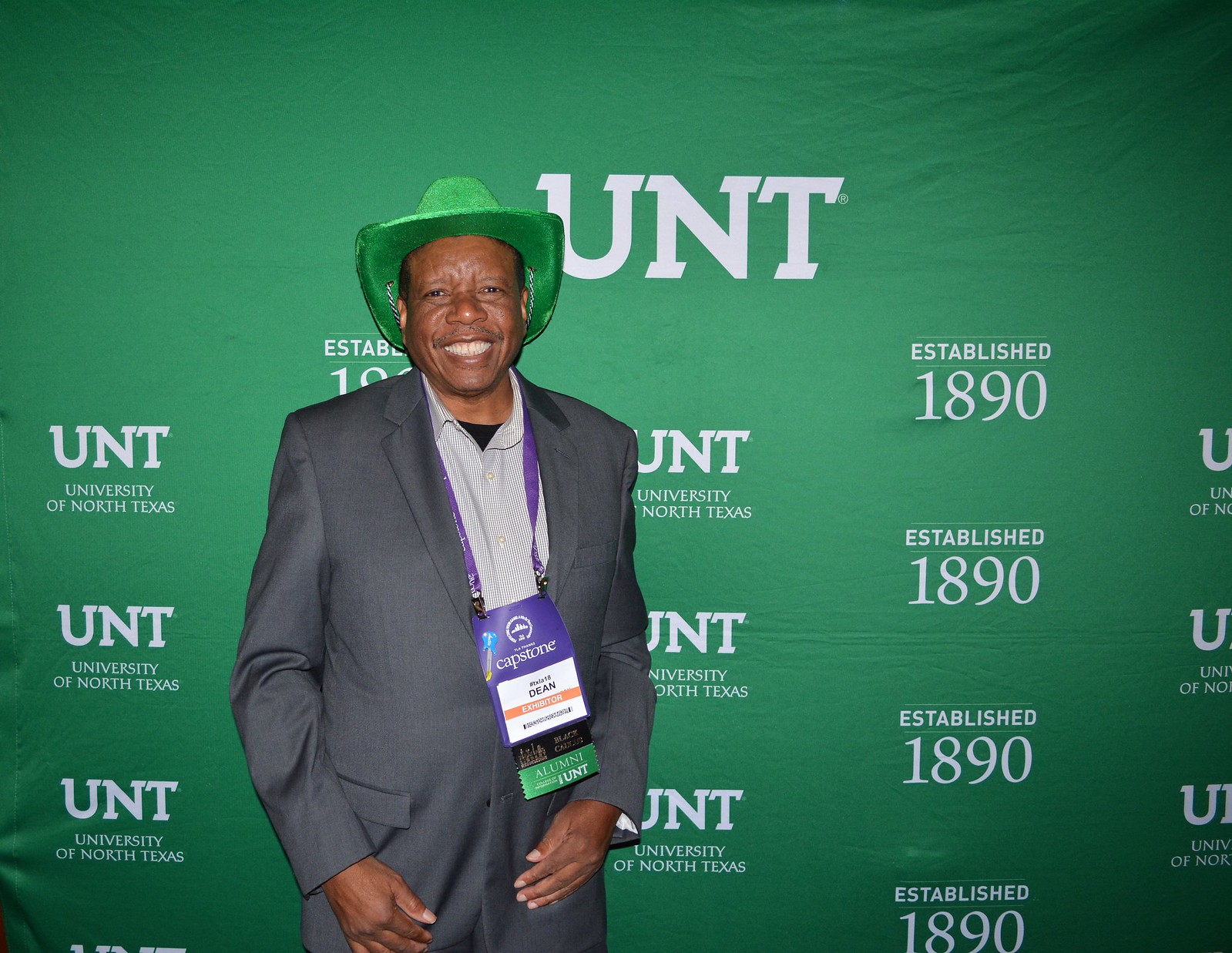This photograph features an older black man standing and smiling in front of a green backdrop adorned with white text. He is attired in a green cowboy hat, dark gray suit jacket, light blue button-down shirt, and a black t-shirt. Around his neck, he wears a lanyard with an ID badge that identifies him as "Dean," an exhibitor and alumni from the University of North Texas (UNT). The backdrop behind him is repetitive, displaying the phrases "UNT," "University of North Texas," and "Established 1890" numerous times in white lettering. Dean appears joyful and proud, likely attending an alumni event at his alma mater.